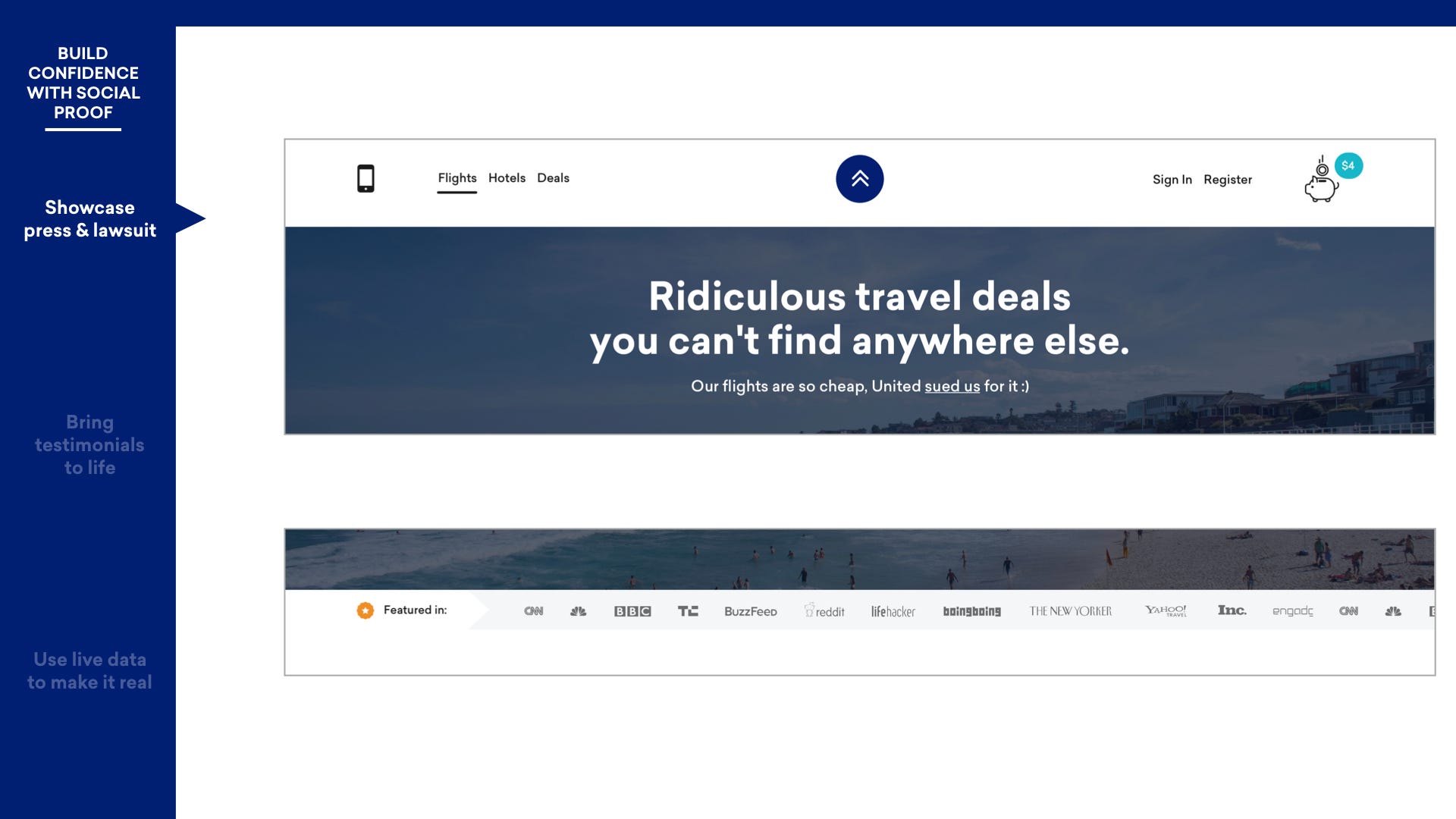This is a detailed screenshot from a travel website. On the left side, there is a blue vertical rectangle with white text that reads, "Build confidence with social proof. Showcase press and lawsuit, which is selected. Bring testimonials to life. Use live data to make it real."

To the right, there is a white area. At the top of this section, tabs labeled "Flights" (selected), "Hotels," "Deals," "Sign In," and "Register" are presented. An icon of a piggy bank with a coin dropping into it is featured, with a blue circle to the right displaying "$4" in white lettering.

Beneath this, a banner announces, "Ridiculous travel deals. You can't find anywhere else. Our flights are so cheap, United sued us for it. :)" The background image showcases a bustling beach with numerous people engaged in various activities. The waves are visible on the left side of the image, with houses seen in the distant background.

At the bottom, a list of media outlets where the website has been featured includes CNN, NBC, BBC, TLC, Buzzfeed, Reddit, Lifehacker, Boing Boing, The New Yorker, Yahoo Travel, INC, and ENGADC. The list then begins to repeat, starting with CNN and NBC again.